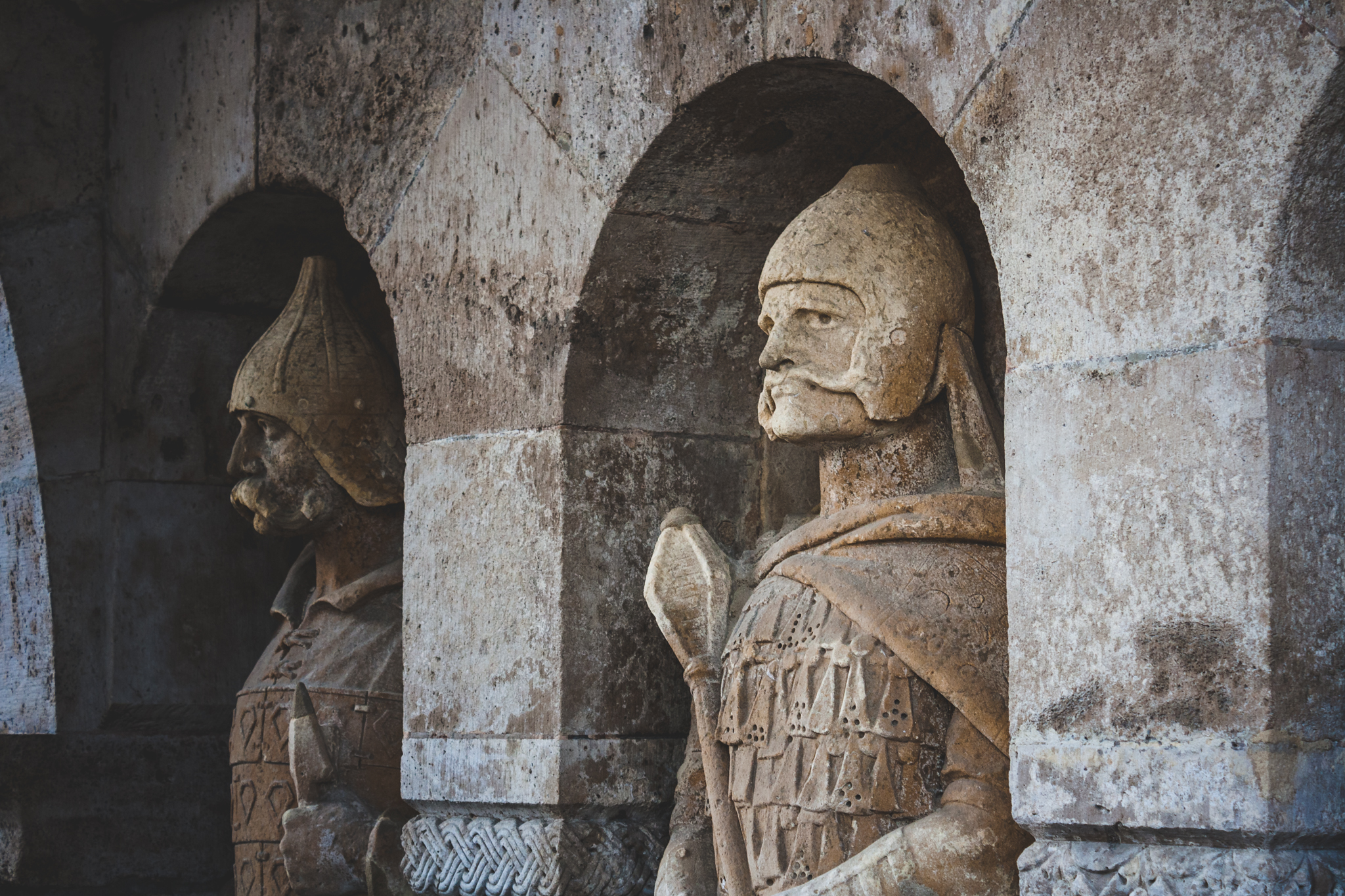The photograph showcases two aged, sculpted figurines positioned within small arch-shaped alcoves that resemble castle walls. These statues, each fitting comfortably inside their respective alcoves, depict formidable soldiers. Carved from cement or clay that has faded to hues of grayish light orange, the material bears the marks of time with visible stains. Each soldier is equipped with distinct weapons: the left figurine holds a spear resting on the ground in its left hand, while the middle figurine is designed gripping a mace. Both statues feature elaborate details, including helmets, chainmail chestplates adorned with tiny, thin triangles, cloaks draped over their shoulders, and arm guards. Their faces are marked by mustaches, the left soldier with a thick mustache, and the one in the middle with a thinner variation, both peering intently to the left.